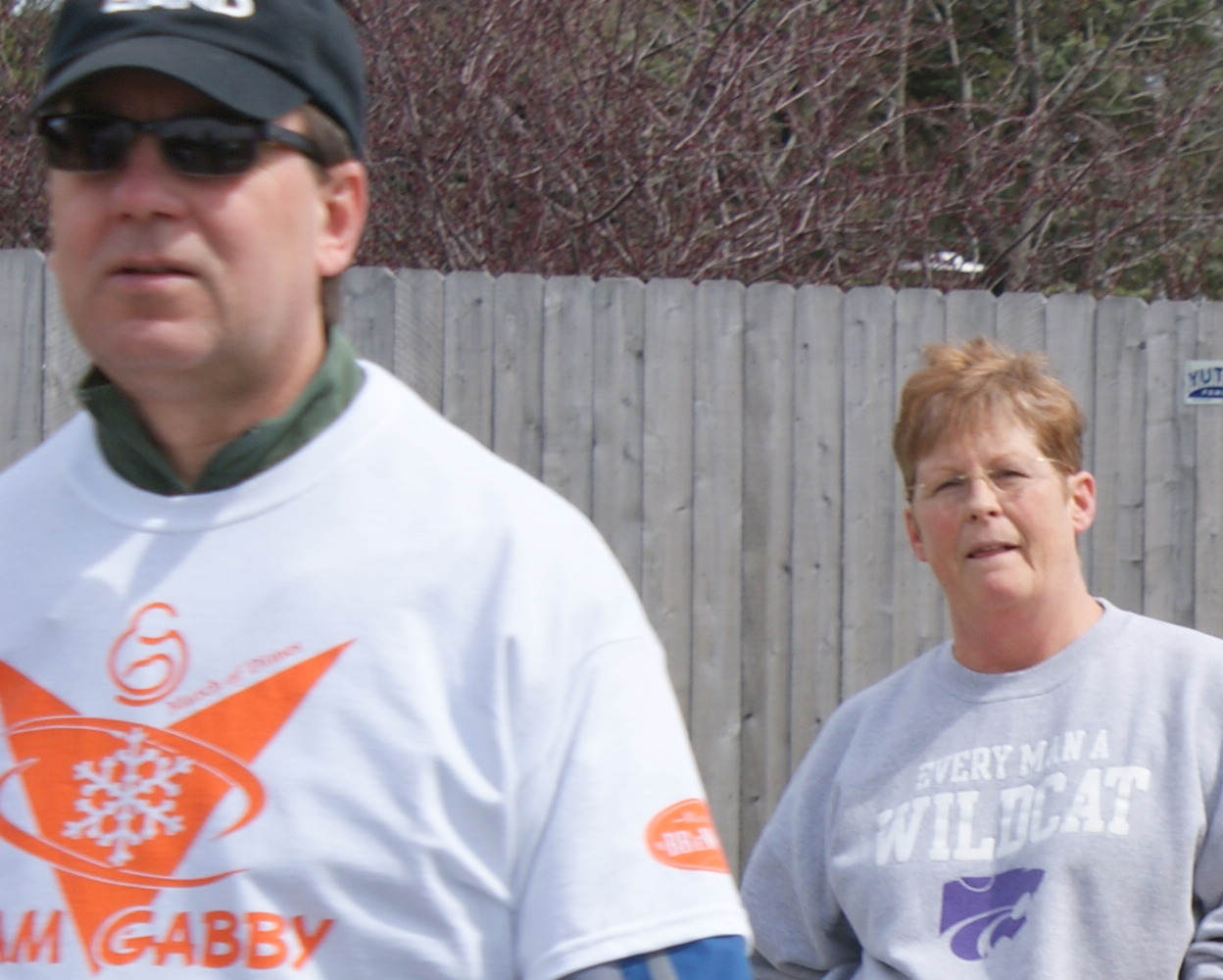In this full-color outdoor photograph, a man and a woman, both appearing to be middle-aged, are positioned in front of a large wooden fence with leafless trees visible in the background, suggesting it's either late fall or winter. The man, who seems to be positioned slightly in front of the woman and closer to the camera, is wearing a black hat, sunglasses, and a white shirt with orange text that partially reads "GABBY." The shirt also features an emblem resembling an upside-down triangle with a white snowflake in the middle, and a green shirt is visible underneath the collar. The woman, standing to the right of the man and slightly behind, has very short brown hair and is wearing reading glasses. She is looking directly at the camera and dressed in a gray sweatshirt with the text "Every Man a Wildcat" and a purple drawing of a wildcat below.